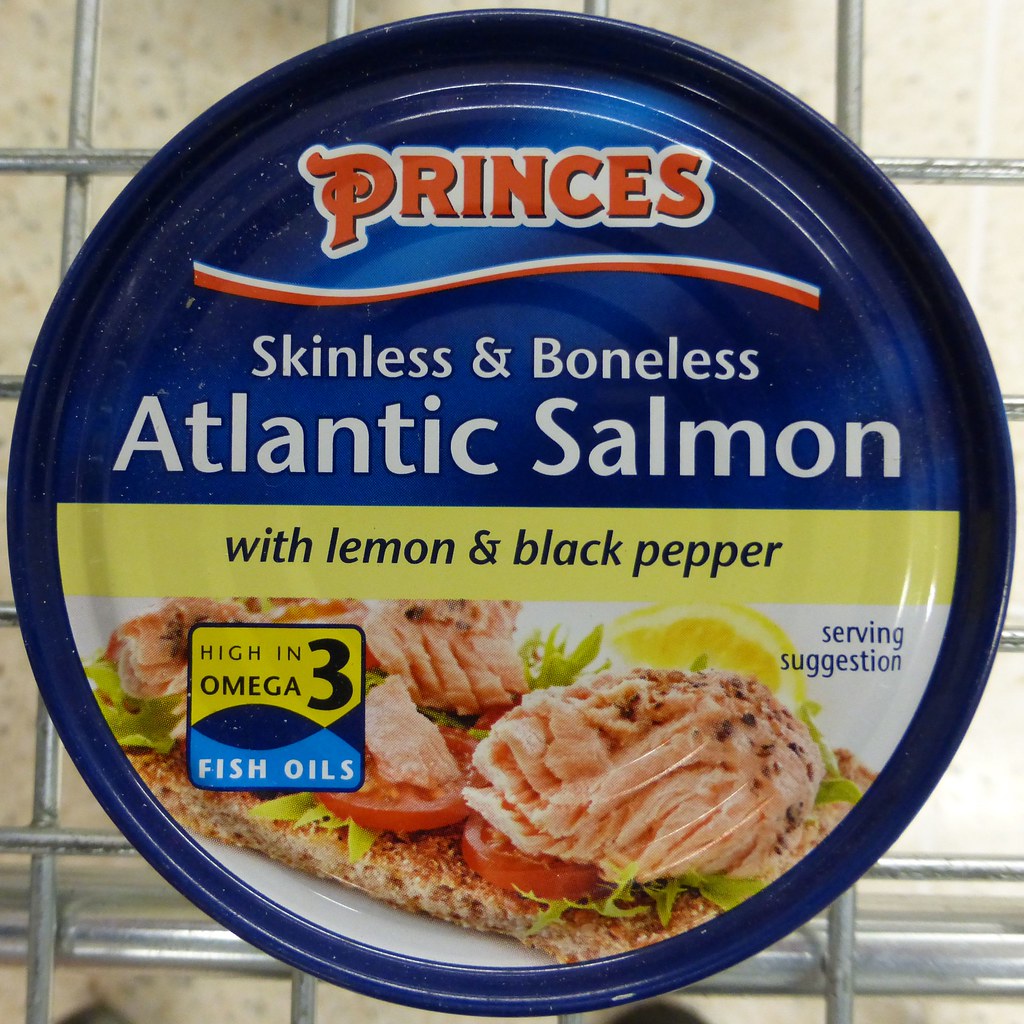This square image features an overhead shot of a can of skinless and boneless Atlantic salmon. The can itself is a blue, metal container with detailed labeling. At the top, the brand name "Princes" is displayed in bold red letters outlined in white. Directly beneath this, a wavy line of white and red separates the logo from the product description. The text "skinless and boneless Atlantic salmon" is written in white letters against the blue background. 

Further down, a yellow bar spans the lower portion of the label, containing the text "with lemon and black pepper" in navy blue lettering. Beneath the text is an appetizing image of flaked salmon placed atop a slice of bread, garnished with tomatoes and some vegetables. The background of the image features a slice of lemon and a serving suggestion on a white surface. Additionally, a note about the product being high in omega-3 fish oil is included.

The can is placed inside a shopping cart, viewed through standard gray steel bars, with what appears to be a white concrete surface visible below.